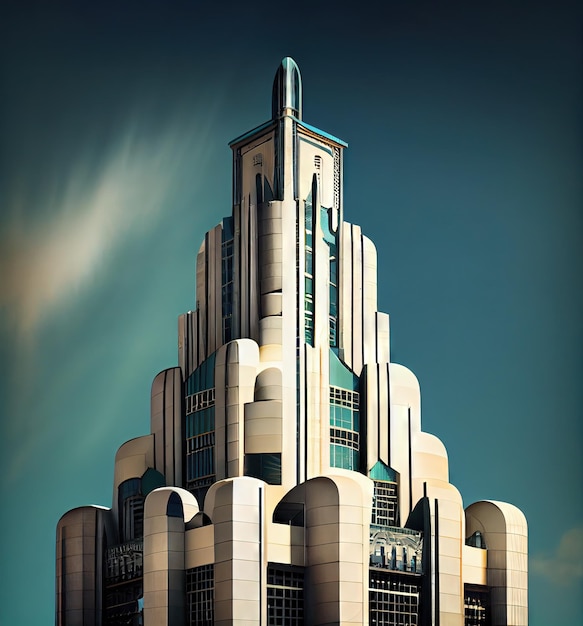The image depicts the top of an Art Deco-style building with distinct terraced, triangular architecture that narrows as it ascends, culminating in a rocket-like tip. The structure is constructed primarily of beige bricks with light greenish-blue accents that match the sky's hue. Sunlight illuminates the right side of the building, casting shadows on the left. The façade features plenty of windows, and the design includes large, rounded granite blocks, adding to its robust appearance. The sky behind the building transitions from muted indigo blues in the upper right corner to lighter, greenish-blue tones in the lower left, with wispy clouds that appear smudged upwards. The overall scene has a digital, possibly AI-generated feel, accentuated by the precise and vivid architectural elements.